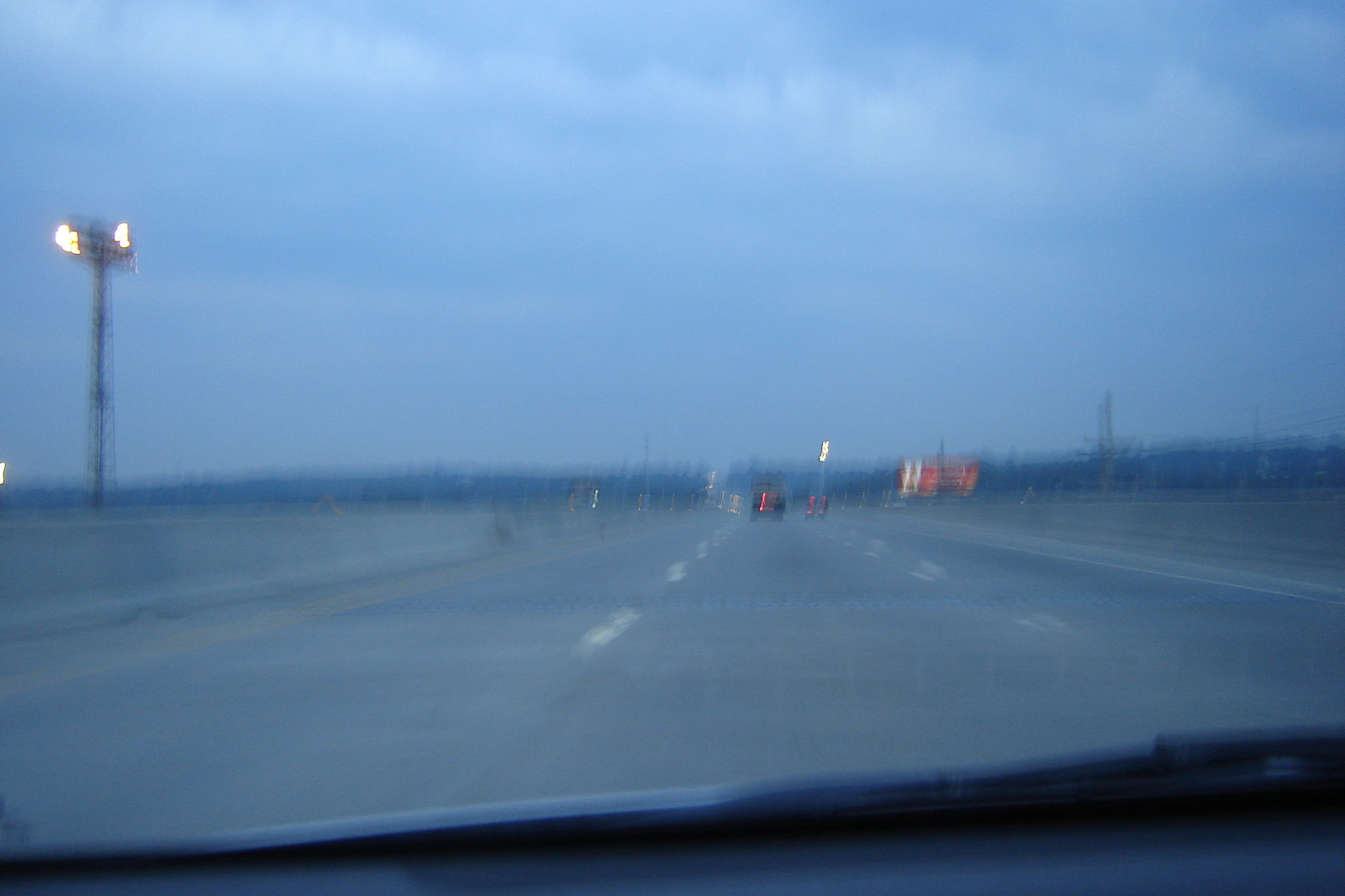A very blurry image taken from inside a moving car on a three-lane highway. The shot reveals part of the dashboard and windshield wiper, suggesting the photo was captured from the passenger side. The highway, obstructed by a concrete divider on both sides, reveals only a few scattered cars in the distance, their bright red taillights gleaming against the dim surroundings. It appears to be nearing dusk or heavily overcast, casting a dark blue-gray hue over the scene. On the left, a towering streetlight, reminiscent of those in football stadiums, stands out, while on the right, several power poles flank an indistinct, likely orange and red billboard. In the far distance, a silhouette of dark-colored trees or mountains forms the skyline, underscoring the dreariness of the day.